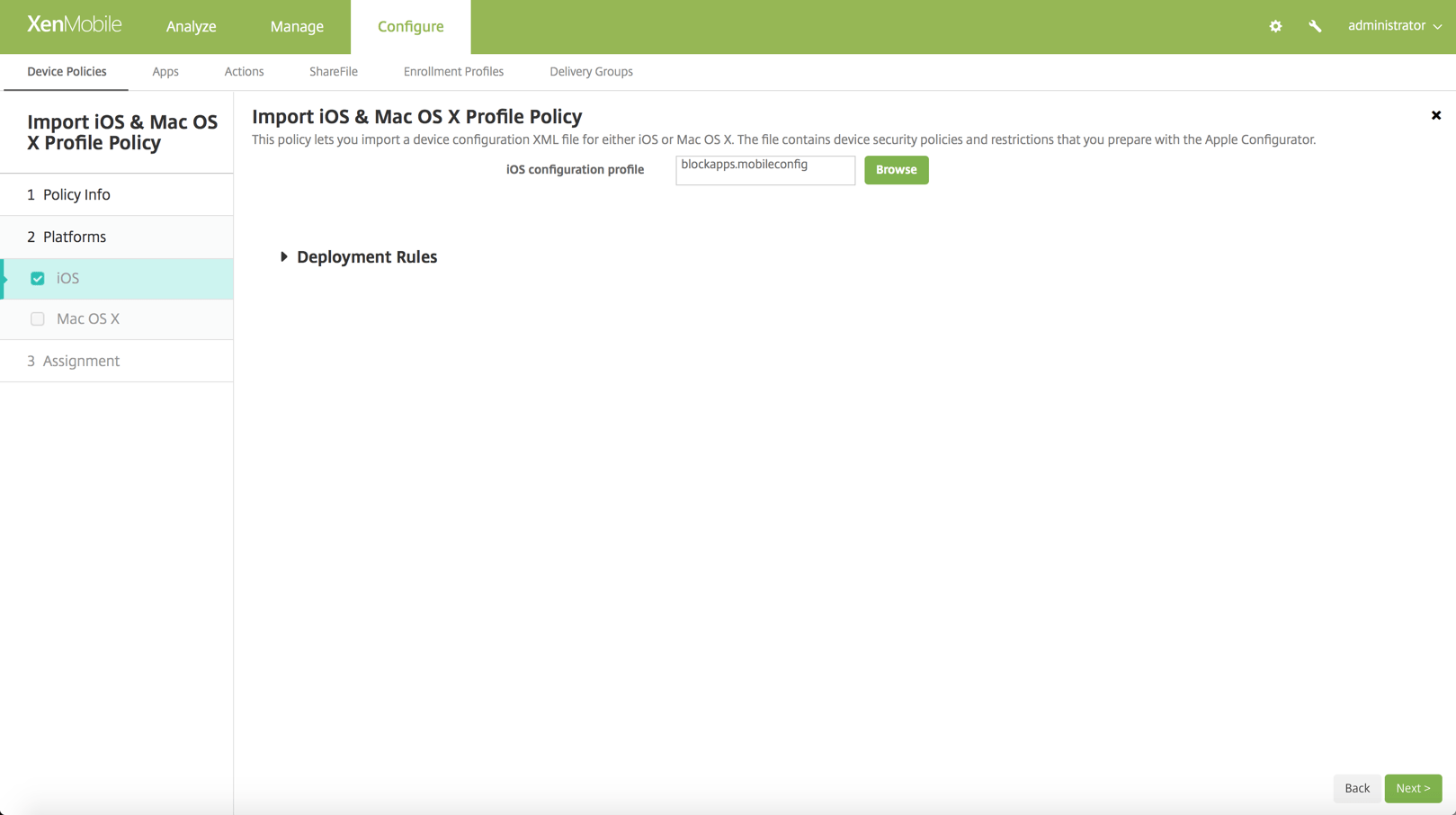This screenshot primarily features a clean, white interface. At the top, there is a light green bar with white text displaying various options: "ZenMobile," "Analyze," "Manage," "Configure," along with a gear icon, a tool icon, and the text "administrator" with a drop-down menu. The "Configure" tab is highlighted.

Directly below this top bar is another navigation bar in white with dark text, presenting the following options: "Device Policies," "Apps," "Actions," "Share Files," "Enrollment Profiles," and "Delivery Groups," with "Device Policies" currently selected.

Further down, a third menu is visible with bold text stating "Import iOS and MacOS X Profile Policy" and three listed items underneath: "1. Policy Info," "2. Platforms," and "3. Assignments," with "Platforms" currently selected.

On the right side of the screen, there is sparse text surrounded by a lot of white space. The text reiterates "Import iOS and MacOS X Profile Policy" and includes a designated area for "iOS Configuration Profile" with a "Browse" button, along with a menu for "Deployment Rules."